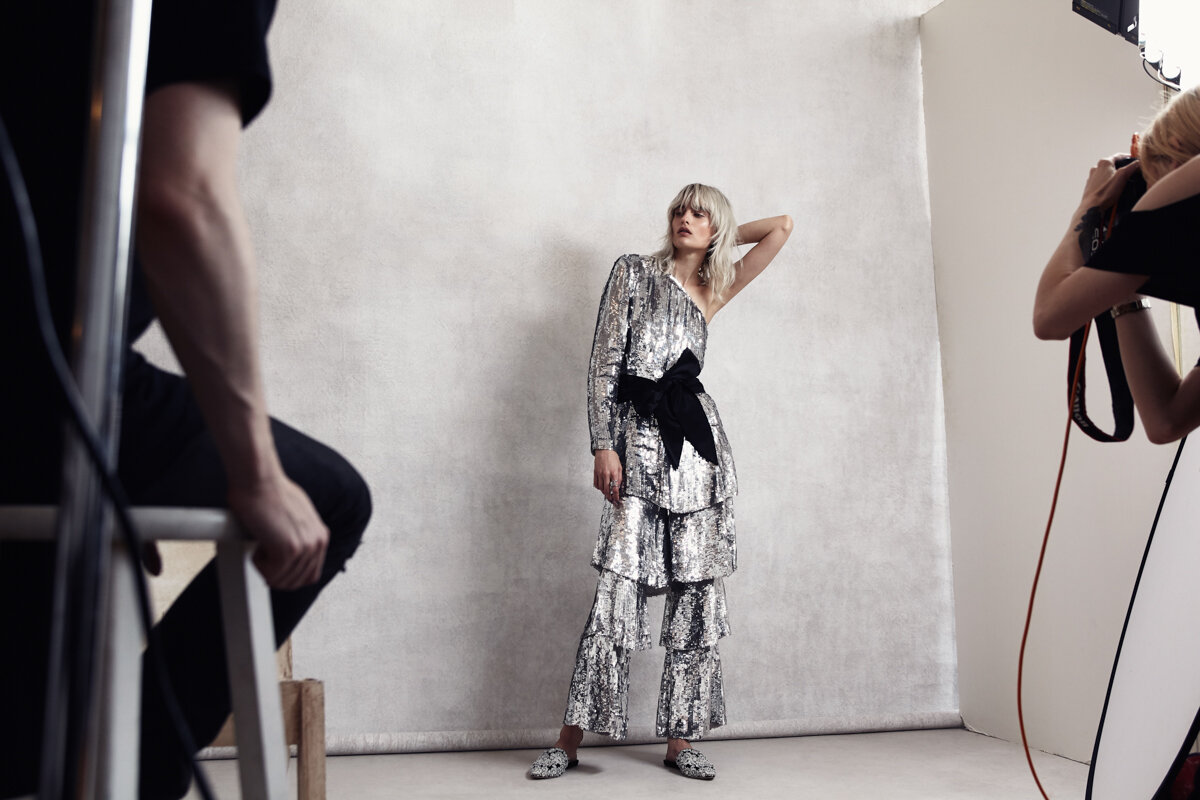In this striking fashion shoot, a model exudes elegance in a sophisticated silver and black ensemble. Her outfit features a one-sleeved design with a long silver sleeve contrasted by a sleeveless side, creating a dramatic diagonal line across her chest. A large black bow cinches her waist, adding a touch of playful femininity. Her look is complemented by matching silver shoes. The pants are uniquely styled, consisting of three layered segments resembling mini skirts for each leg, topped off with a fourth layer that drapes down from the waist to the thigh, mimicking a dress overlay.

She poses against a subtle white and light gray background, emphasizing the complexity of her outfit. Her blonde hair adds a soft contrast to the bold fashion statement. In the foreground, a man dressed entirely in black—shirt and pants—sits on a stool, his arm visibly holding onto it. Towards the right upper corner of the image, studio equipment such as tungsten photography lights and a blurred blonde photographer with a camera is visible. The photographer sports a stylish black short-sleeved shirt with a noticeable shoulder cut-out. Two wires snake down to the bottom of the frame, indicative of an active and dynamic studio environment.